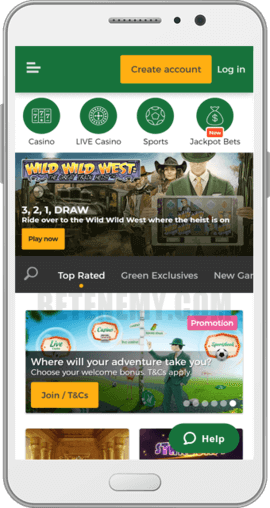The image showcases a front-facing view of a smartphone, set against a white background. The phone itself has a realistic silver frame with curved corners and a speaker at the top, although it might have been digitally rendered in 3D. 

In the center of the screen, a mobile app interface, which appears to be for a gambling website, is displayed. The top of the screen features a green bar containing a white menu icon on the left, a "Create Account" button with black text on a golden-yellow background and rounded corners in the middle, and a white "Login" link to the right.

Below the green bar, the background shifts to white, where there are four circular icons. Each icon represents a different section of the app:
1. The first icon, labeled "Casino," features an illustration of a slot machine.
2. The second icon, labeled "Live Casino," displays a circle icon with a cross inside it.
3. The third icon, labeled "Sports," shows a soccer ball.
4. The fourth icon, labeled "Jackpot Bets," features a money sack and a red rectangle badge that says "New."

The main body content begins with a promotional header titled "Wild Wild West," depicting illustrated cowboys and a cowgirl holding a tablet. The header text reads, "Three, two, one, draw! Right over to the Wild West where the heist is on. Play Now," accompanied by a yellow button.

Below the header lies what appears to be a submenu. It includes a search icon and the text "Top Rated" in white, with a yellow dot indicating the active section. To the right are additional sections: "Exclusives," labeled in green, and "New Games," partially showing as "New GA."

Further down, another promotional banner appears, asking, "Where will your adventure take you?" It depicts a person in a suit standing next to a sign with multiple directions. The promotion text includes "Join" and "TNC's" on a button.

The image also bears a barely visible watermark reading "retenemy.com," centrally placed and spanning across the app's content but not obscuring any specific elements.

Overall, the detailed description of the smartphone screen app offers a comprehensive preview of the gambling website's mobile interface.